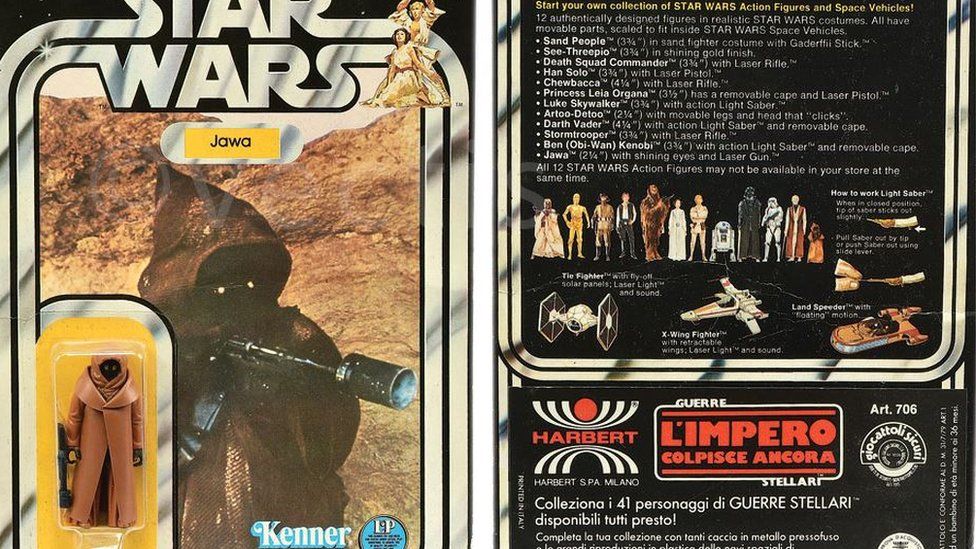This image depicts retro packaging for a Star Wars action figure, likely from the 70s or 80s. The front of the packaging prominently features the Star Wars logo in white letters against a black background. It showcases a Jawa, a small brown-cloaked figure with glowing eyes, holding a gun in its left hand. The Jawa action figure is encased in a clear plastic bubble. Below the character image is the name "Jawa" and the manufacturer's label, Kenner. The left side highlights the figure, capturing the nostalgic essence of vintage toy design. The back of the packaging lists various other Star Wars characters and space vehicles available in the collection. The text encourages fans to "start your own collection of Star Wars action figures and space vehicles." White fonts on a black background describe the licensing details and highlight additional characters, such as L'Imperio, Calypso, and Korra. The design and presentation of this packaging evoke the excitement of assembling a comprehensive Star Wars action figure collection.